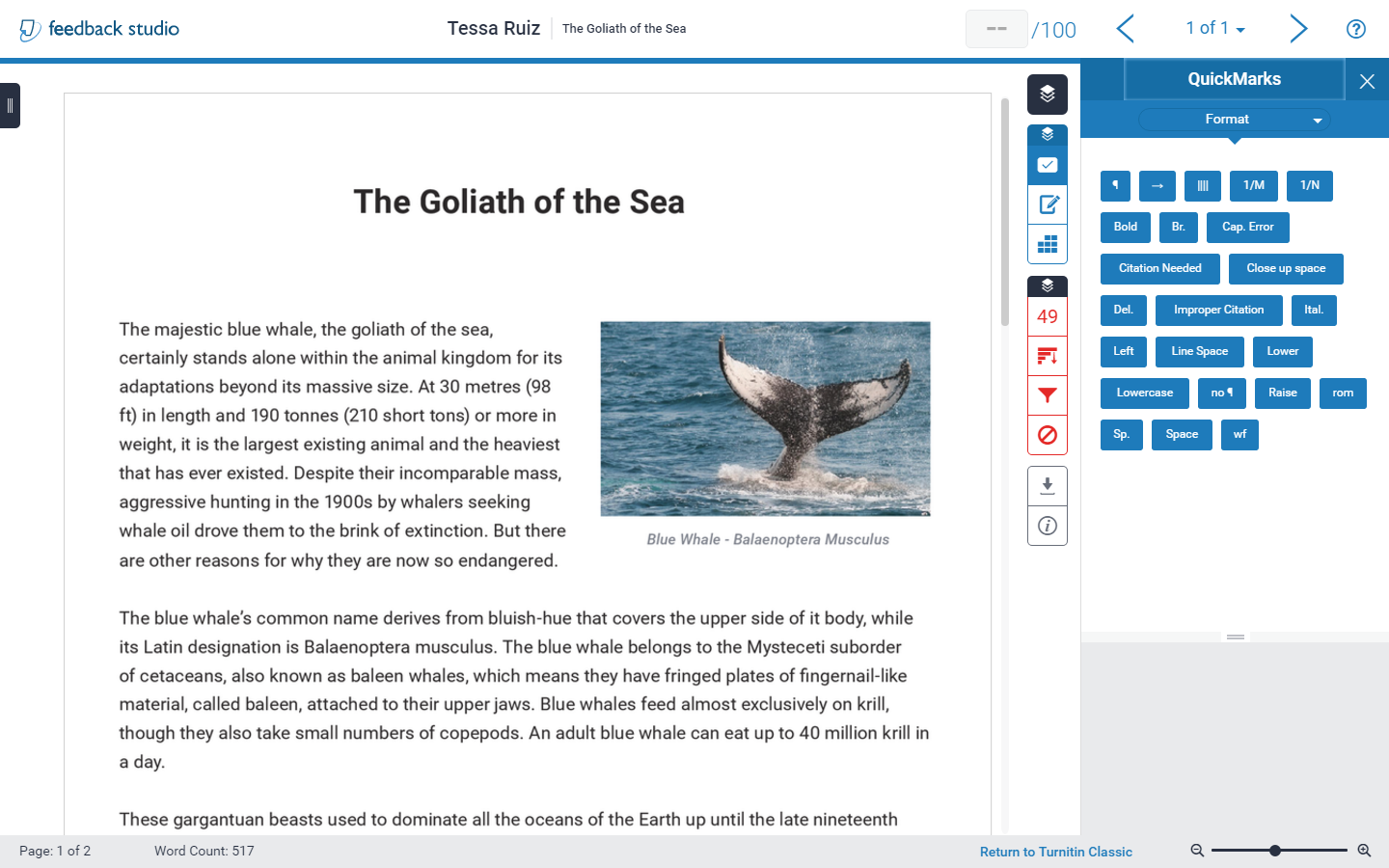At Feedback Studio, a display prominently features the name "Teresa Ruiz" with the title "Goliath of the Sea." Below this, an in-depth article discusses the majestic blue whale, including a striking photograph of a whale's tail emerging from the ocean. The article is titled "The Goliath of the Sea" and delves into the fascinating biology and history of the blue whale (Balaenoptera musculus).

The text highlights the extraordinary size of the blue whale, noting that these magnificent creatures can reach lengths of up to 30 meters (98 feet) and weigh as much as 190 tons (210 short tons). This makes them not only the largest existing animals but also the heaviest creatures to have ever existed on Earth.

The caption explains the blue whale's current endangered status, attributing it largely to aggressive hunting practices in the 1900s when whalers hunted them for their valuable whale oil. Various other factors also contribute to their endangered status today.

The article describes the origins of the blue whale's name, both common and scientific. The common name arises from its distinctive bluish hue that colors the upper side of its body. Meanwhile, its Latin name, Balaenoptera musculus, places it within the suborder Mysticeti. This detailed exploration underscores the unique adaptations and monumental presence of the blue whale within the animal kingdom.